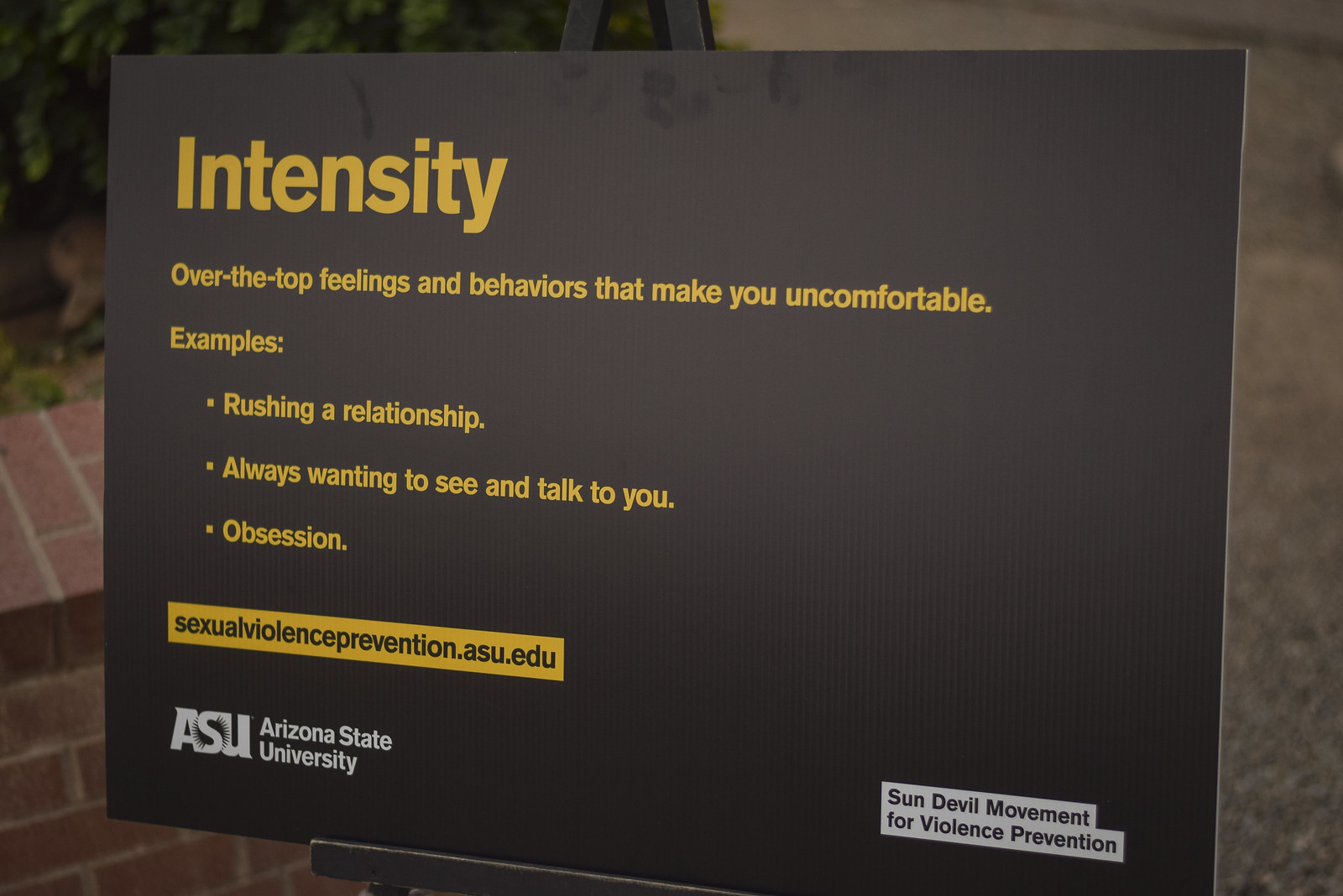The photo captures a sign displayed outdoors, positioned on a black easel against a backdrop that includes red brickwork to the left and concrete or gravel on the ground. The sign is black with white and yellow text, and it appears to have greasy fingerprints at the top, particularly in the middle area. The topmost and most prominent text on the sign, in bold yellow, reads "Intensity." Below this, in smaller yellow letters, it states: "Over-the-top feelings and behaviors that make you uncomfortable." This is followed by the word "Examples:" in yellow, and then a bulleted list in white text that includes: "Rushing a relationship," "Always wanting to see and talk to you," and "Obsession." Further down, there is a yellow rectangular bar with black text that reads "sexualviolenceprevention.asu.edu." In the bottom left corner, the ASU (Arizona State University) logo is displayed in white, and the bottom right corner reads "Sun Devil Movement for Violence Prevention" in white text. The setting includes plants housed within the brick area, and the entire sign setup communicates a message related to sexual violence prevention from Arizona State University.